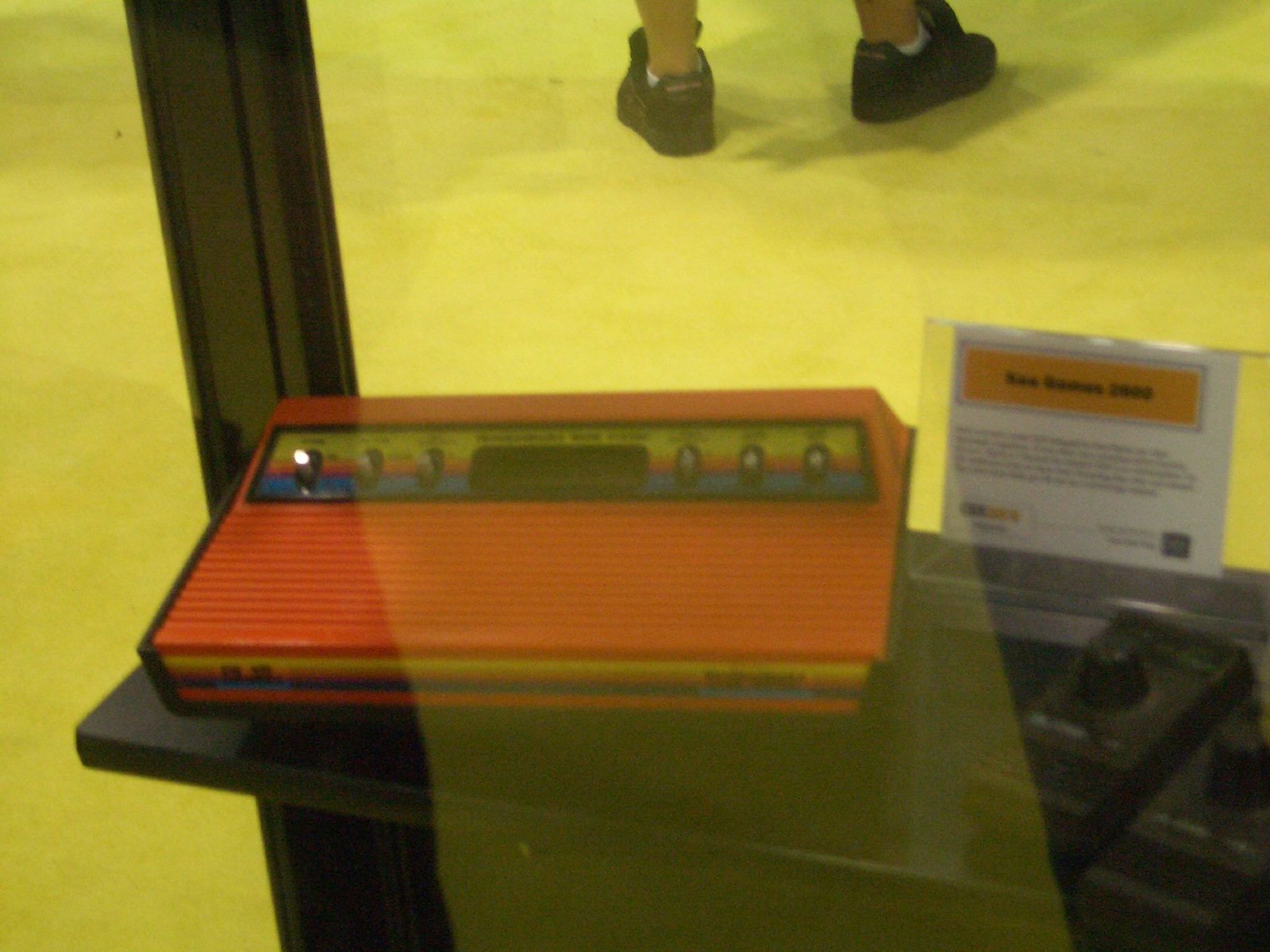The photo depicts a blurry scene with a beige floor and a shelf in the background, featuring an electronic device. In the upper middle towards the right-hand corner, a person's ankles and sneakers are visible. The person has fair skin, is wearing white socks, and mostly black sneakers with indistinct brownish writing on the back. On the shelf, there is a notably bulky and rectangular device, primarily red with yellow and orange stripes. This device, which could be an instrument mix board or a scoreboard, has six metal knobs possibly for volume adjustment. Additional black, bulky remotes are present beside it. Despite the overall yellowish tint and blurry nature of the photo, it hints at the presence of a little sign that might read "see games 2003."